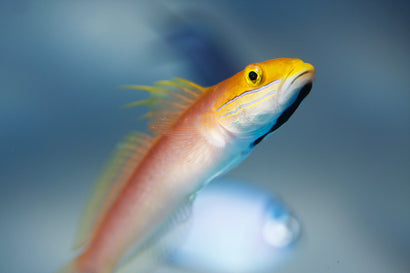This image captures a detailed shot of a beautiful Bella sleeper goby (Valenciennea bella), positioned gracefully at an upward angle from the bottom left corner, centered within the frame. The vibrant fish, elongated and slender, draws attention with its striking coloration: a brilliant yellow crown on its head transitioning to a muted red stripe down its long, luminescent white body. Its dorsal fin is accented with yellow, extending the golden hue from its forehead down the back, which contrasts with its pristine white belly. The fish's eyes are bulging, yellow with black pupils, and beneath its chin lies a distinct thin black stripe. The background is entirely out of focus in a bluish hue, featuring a white and blue orb, possibly another blurred fish, enhancing the foreground fish's sharpness and vividness. This scene offers a stunning portrait of the Bella sleeper goby against a serene backdrop.